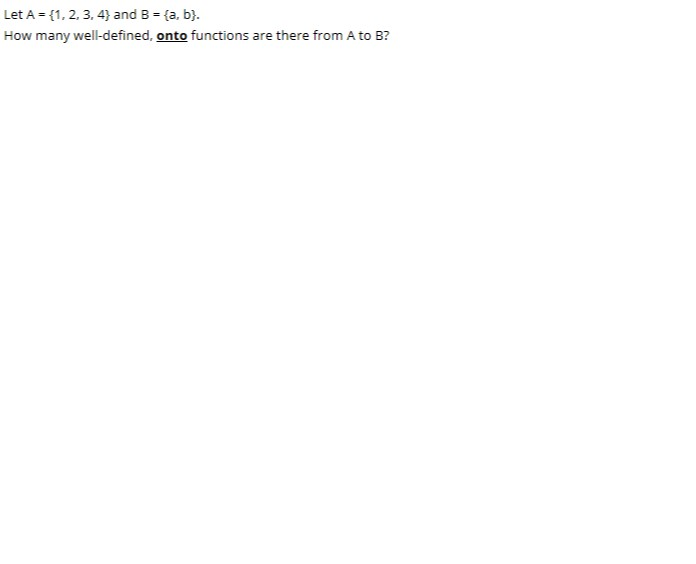The image features a concise mathematical problem presented in black text on a white background, located in the upper left-hand corner. The problem poses a question about onto functions and is formatted as follows:

"Let A = {1, 2, 3, 4} and B = {a, b}. How many well-defined *onto* (where the word "onto" is both bolded and underlined) functions are there from set A to set B?"

The rest of the image is blank white space.